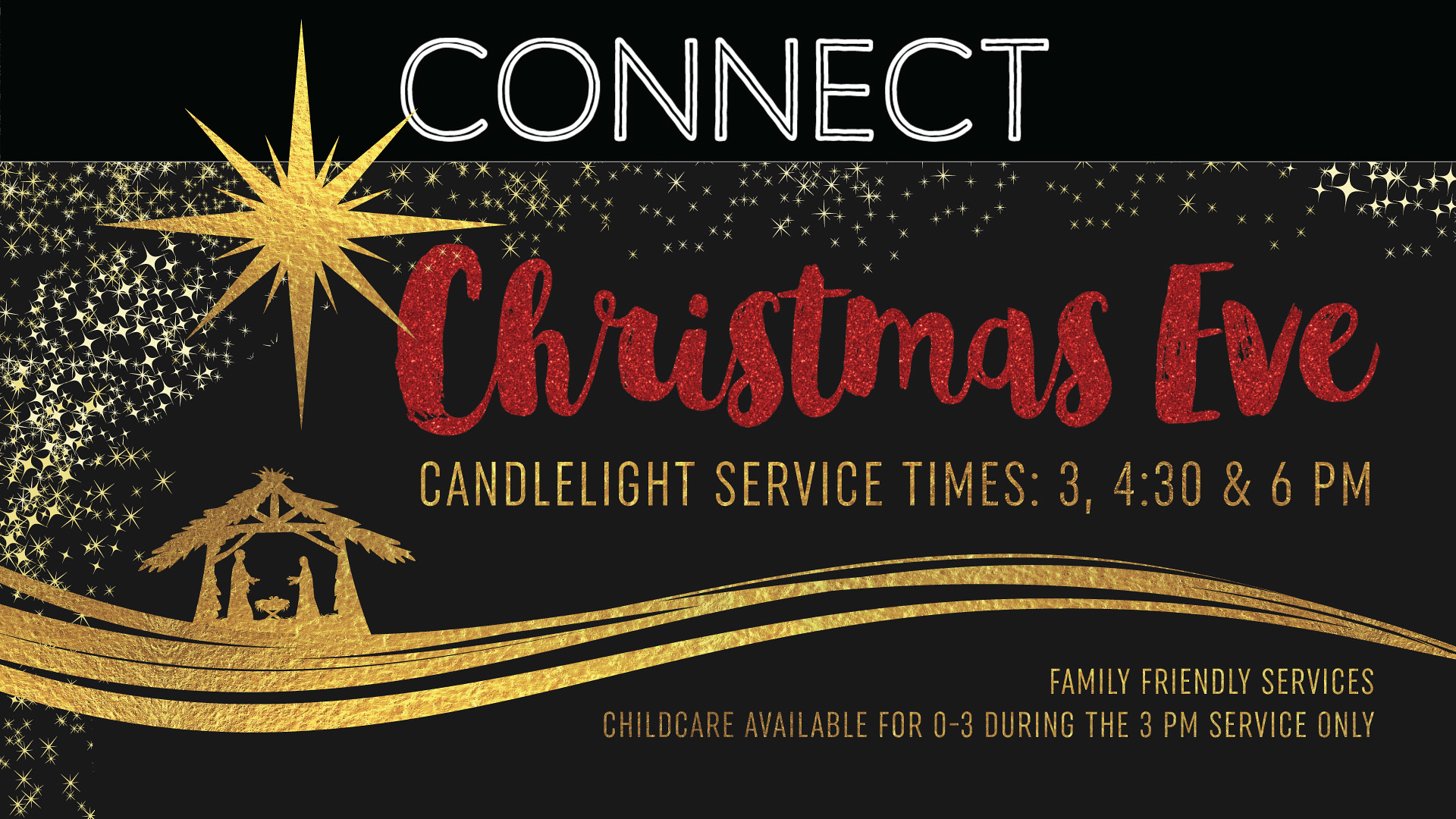The image is a horizontal, rectangular poster advertising Christmas Eve services. The top fifth of the poster features a black header with white text that reads "Connect," utilizing a thin black pinstripe within the letters. Below the header, the background remains dark, accentuating the golden and red elements. In the center, "Christmas Eve" is written in bold, red cursive with a glittering effect. Directly underneath, in gold print, it states "Candlelight Service Times" followed by "3, 4:30, and 6 p.m."

On the left side of the poster, an eight-pointed star and numerous smaller stars in gold lead the viewer's eye downwards and across the top of the image. Below this, there's a depiction of the Star of David positioned above a golden manger scene featuring Joseph, Mary, and baby Jesus. This scene is accentuated by wave patterns flowing from left to right across the poster. 

In the lower right corner, text in gold announces "Family Friendly Services, Child Care Available for 0-3, during the 3 p.m. service only," rounding out the informative and festive design of the poster.